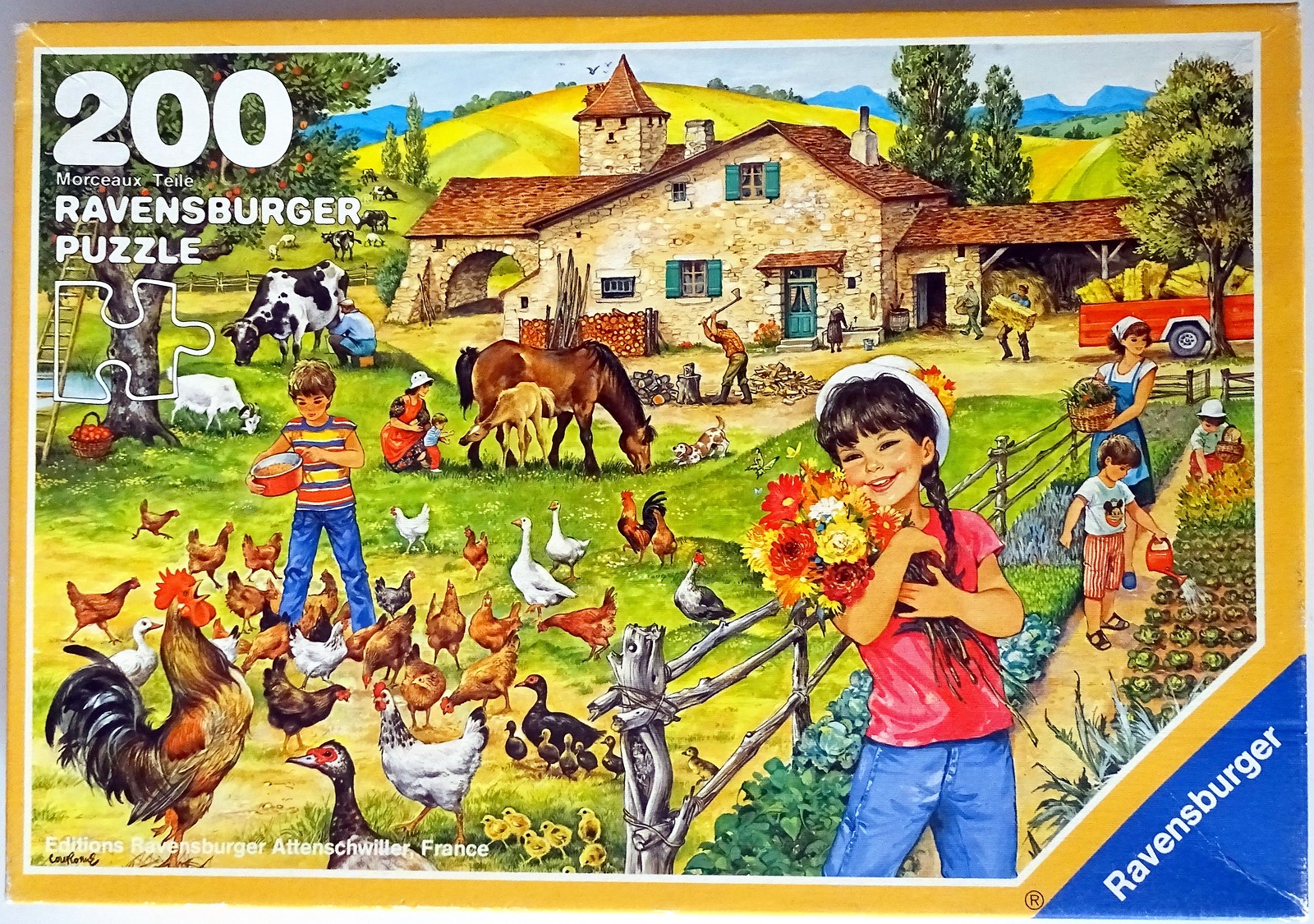The image features the box cover of a 200-piece Ravensburger puzzle. In the bottom right corner, there is a distinctive blue triangle with white text reading "Ravensburger," and a circle containing the letter "R." The box has a yellow border and the words "200 Ravensburger Puzzle" are prominently displayed in the top left.

The illustration on the puzzle cover depicts a lively farm scene bustling with activity. In the foreground, a young boy clad in a Mickey Mouse shirt feeds a large group of chickens with a bowl filled with feed. Beside him, a young girl clutches a bouquet of flowers. Another young child can be seen further back, accompanied by an older woman who is gathering crops into a basket. To the right, a woman guides children as they water plants, which appear to be vegetables like lettuce.

The background reveals a rich pastoral landscape with various elements: a man is seen milking a cow, another chopping wood, and people picking apples from an apple tree. Horses, a cow, and numerous chickens populate the scene, and a barn is visible in the distance. The setting is further enriched by the presence of hills, trees, ducks, a fence, a garden, and vegetables, encapsulating a vibrant, rural atmosphere.